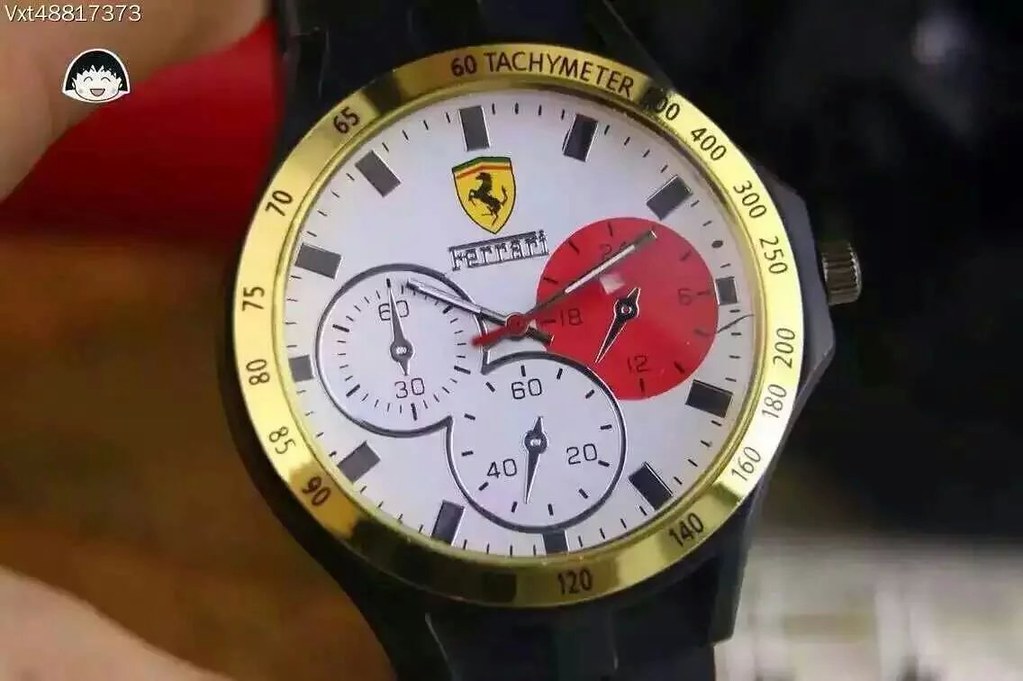This photograph showcases a Ferrari wristwatch with a sleek black wristband and a gold bezel labeled "tachymeter," featuring etched numerals around its circumference. The watch's face is white, adorned with the iconic yellow Ferrari shield logo with a black horse silhouette at the top center, accompanied by the Ferrari name underneath. The primary hands of the watch are black with white stripes, while the second hand is red. Noteworthy details within the face include three sub-dials: one marked at intervals of 60 and 30, another with a scale of 60, 40, and 20, and a third red dial indicating 24, 6, 12, and 18. The hour markers are represented by large black rectangles, and minute indicators are small dashes, providing a modern, minimalist aesthetic. The blurred background highlights the watch's prominent features, with a visible watermark "VXT48817373" in the corner, ensuring focused attention on the intricate design of the wristwatch.